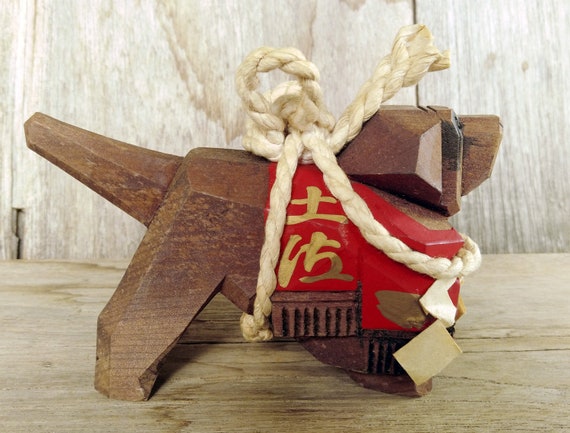This image features a meticulously carved wooden dog, crafted in the likeness of a Tosa Inu, a Japanese breed. The sculpture appears to be assembled from various sized wood blocks, with distinct segments forming the head, body, legs, and tail. The overall color of the wood is natural, though the dog is adorned with a red, vest-like piece, also wooden, that is painted onto its midsection. This red vest features gold characters written in Japanese, which add an element of cultural authenticity.

A thick, off-white rope is tied around the dog's neck, creating an impression that it might be used to lift or perhaps hang the sculpture, although its exact purpose remains unclear. Notably, a tag is visible hanging from the right side of the rope. The entire piece is situated on a sturdy wooden stand or table, enhancing its presentation. Behind the sculpture, a wooden backdrop further emphasizes the natural and rustic aesthetic of the scene. The dog itself is darker in color, contrasting subtly with the lighter wood of the background and stand, bringing the overall composition together in a harmonious display of carved artistry.